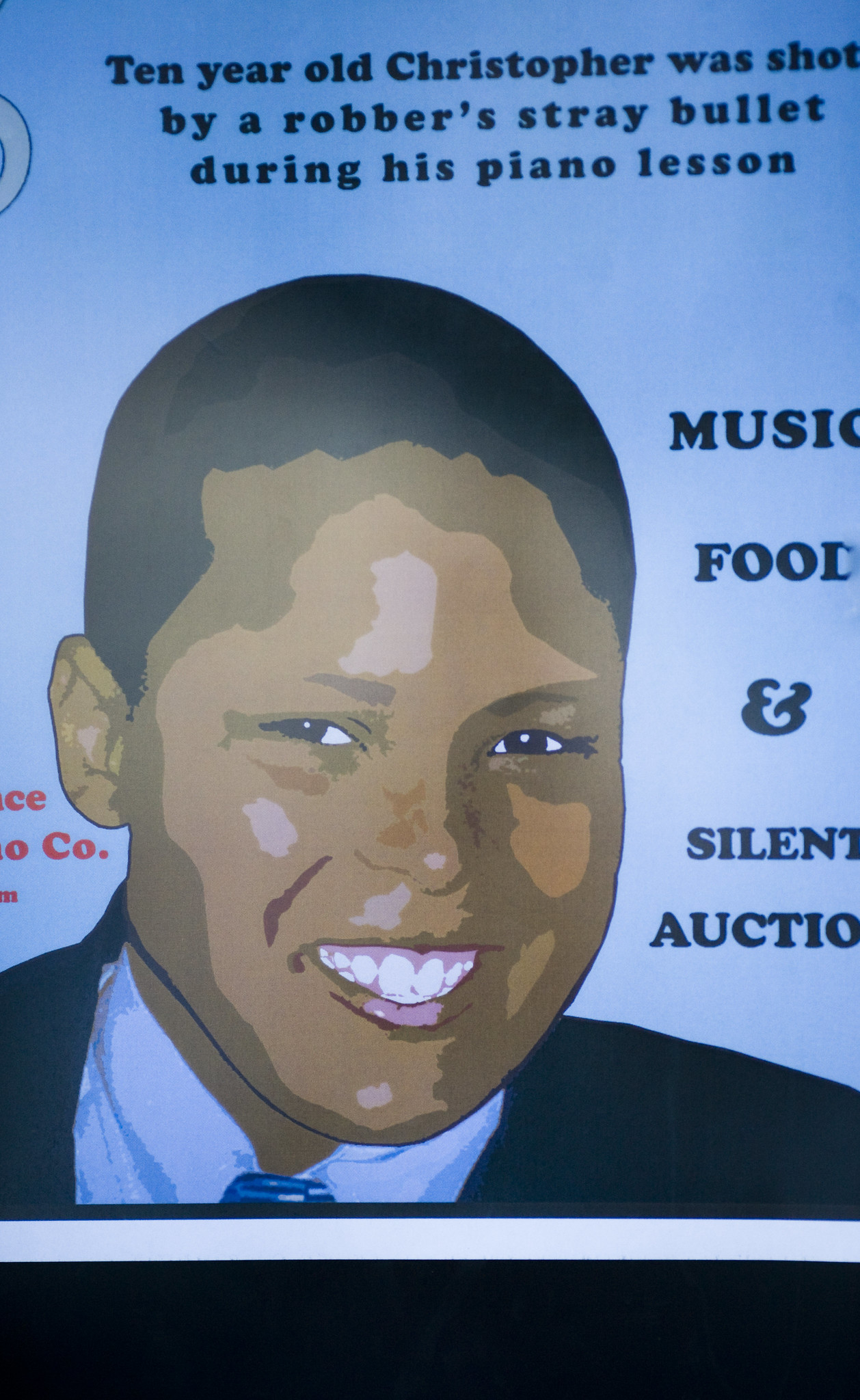This is a detailed description of a poster with a blue background displaying a cartoonized image of a smiling young black boy identified as 10-year-old Christopher. He has short, dark hair, bright white teeth, and pink lips. Christopher is clean-shaven and dressed in a black suit jacket, a light blue shirt, and a blue tie. The top of the poster features black text that reads, "10-year-old Christopher was shot by a robber's stray bullet during his piano lesson." To the right of Christopher's image, additional text in dark blue capital letters announces "Music, Food, and Silent Auction." The image is truncated on the sides, making some red-colored text partially visible near his ear on the left side, with letters like "CE" at the top and "O, C" or possibly a dot below it, suggesting other texts that are not fully readable. The bottom part of the poster is black. This poster appears to be promoting a fundraiser, likely to support or cover expenses related to the tragic event involving Christopher.